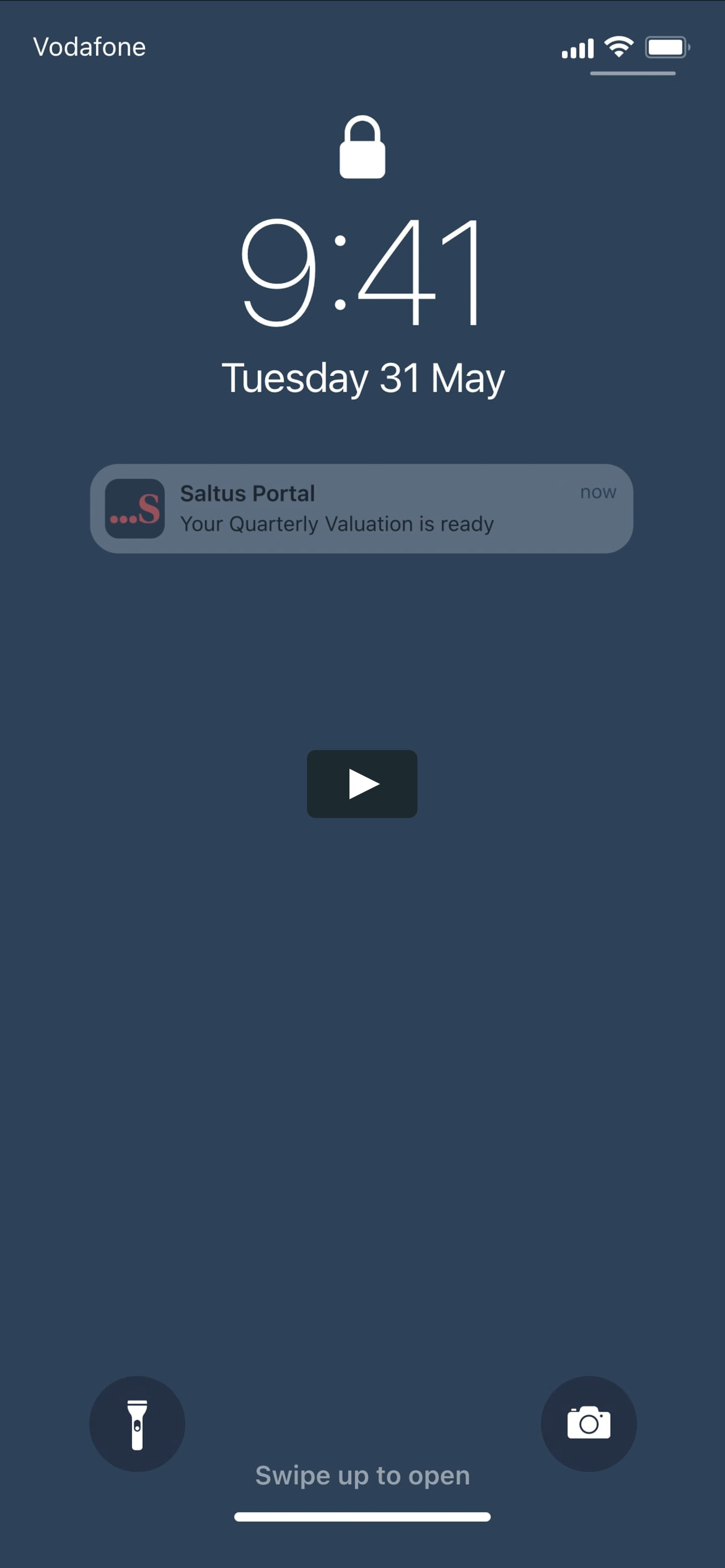A detailed caption for the described image is as follows:

"This image portrays the lock screen of a smartphone belonging to a Vodafone network user. The lock screen features a sophisticated grayish-blue background. In the top left corner, the carrier name 'Vodafone' is prominently displayed in white text. Adjacent to this, signal strength bars, a Wi-Fi icon, and a fully charged battery icon, depicted as a white-filled battery lying horizontally, can be seen. Below this information is a thin line separating the notification area.

Centered on the upper half of the screen is a white lock icon, signifying that the phone is locked. Dominating the middle of the display, the time is prominently shown as '9:41' in large, bold numerals. Just below the time, the current date 'Tuesday, 31 May' is written in smaller font.

Further down, a notification panel reads 'status portal' followed by 'Your quarterly valuation is ready.' This message is stamped with a timestamp 'now', concluding with three red dots and an upper-case letter 'S' as part of the notification formatting."